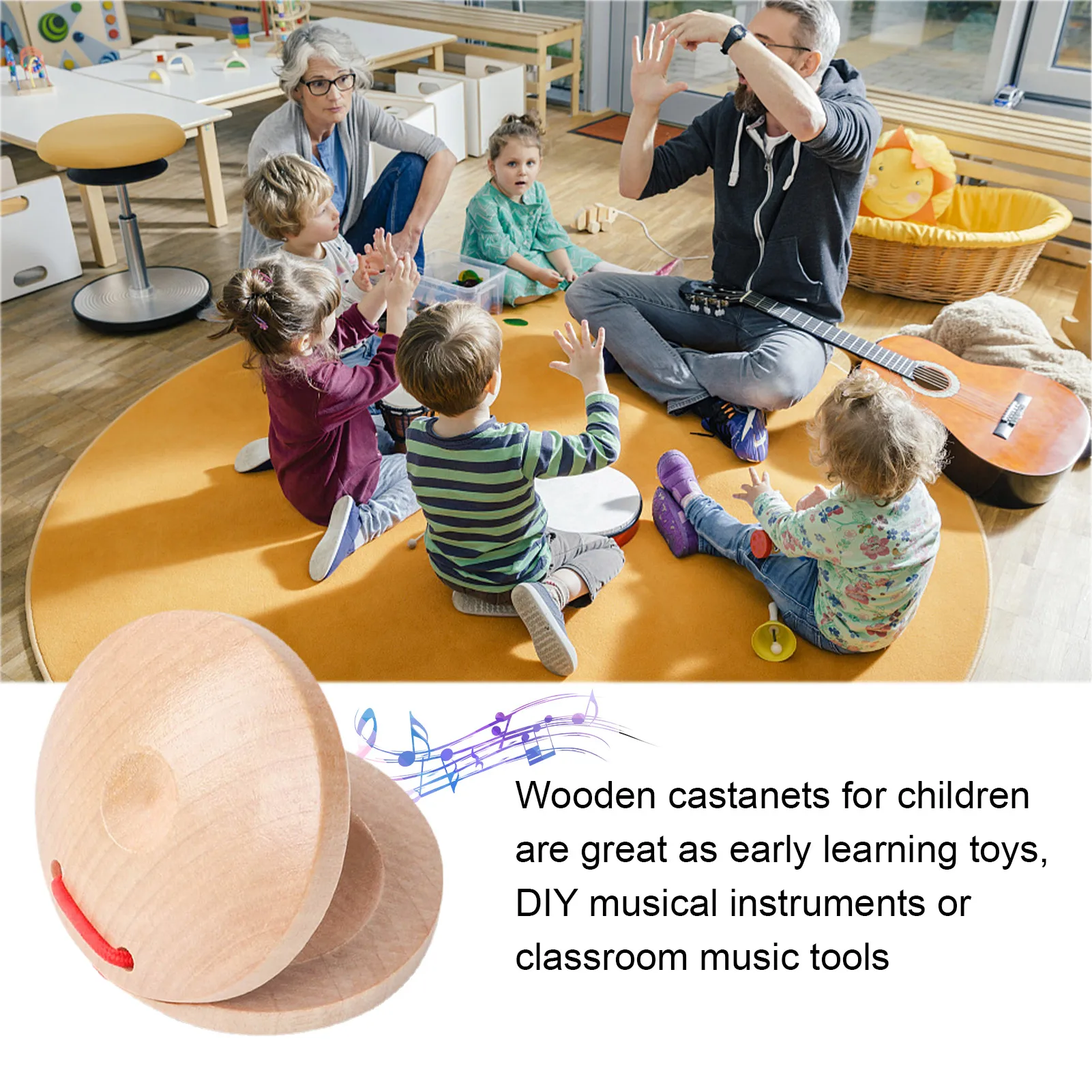This advertisement features a vibrant, well-lit daycare center showcasing a group of children sitting in a circle on an orange mat, along with two adults. One of the adults, a man with a guitar positioned on his lap, appears to be the instructor, while an older woman in a gray sweater sits amongst the children, observing their activities. The children and adults are in a sunny room with wooden flooring, surrounded by little tables and a basket with a pillow, hinting at a creative and inviting learning environment.

Above this scene, the text "Wooden castanets for children are great as early learning toys, DIY musical instruments, or classroom music tools" is prominently displayed. Below this phrase, an image of smooth, light-colored wooden castanets with a red rope handle is shown. The castanets have a clamshell design and emit colorful musical notes in shades of blue and purple, emphasizing their musical function. This detailed advertisement effectively combines the visual appeal of the castanets and their educational purpose.